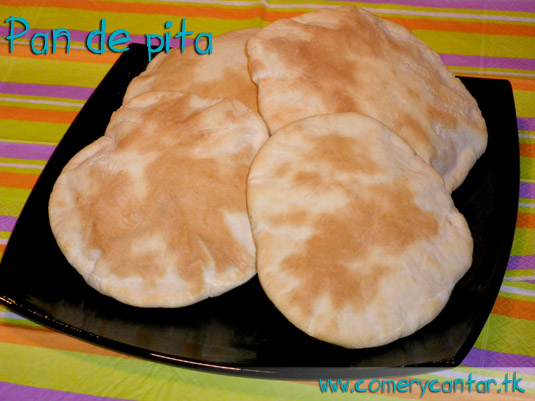In this detailed image, a black square plate is positioned at the center on top of a vibrant striped tablecloth featuring alternating stripes of green (or potentially yellow), purple, and orange. The plate holds four pieces of pita bread, which are round, tan, and slightly charred, displaying a dark golden color. The pitas are stacked and overlapping neatly in the middle of the plate. In the top left corner of the image, the text "Pan de Pita" is written in light blue letters. At the bottom of the image, a web address, www.comerycantar.tk, is prominently displayed, indicating a recipe site or restaurant.